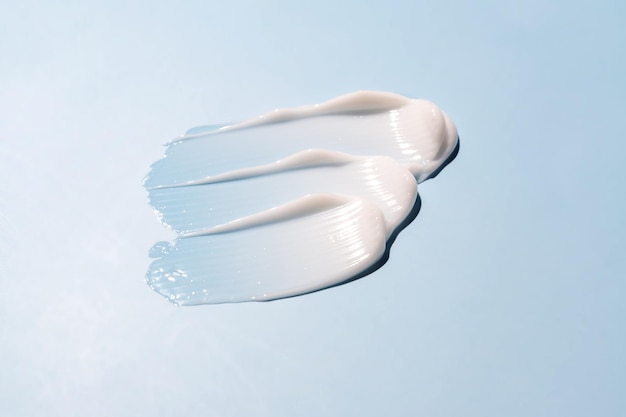The image showcases three distinct swatches of a pale paint or lotion on a light blue background. Each swatch starts on the left as a medium blue and transitions to a lighter blue, ultimately becoming almost off-white by the right edge. Arranged one behind the other, these swatches are created by either a paintbrush or a makeup applicator, as indicated by their ridged texture and curved edges. The strokes are thicker on the right, subtly casting shadows to the right, indicating a light source from the left. The overall effect is one of smooth, shiny, and slightly thick strokes that have a gradual color gradient and a clear separation between each one. There is no text or other elements in the photo to distract from the three visually striking swatches.